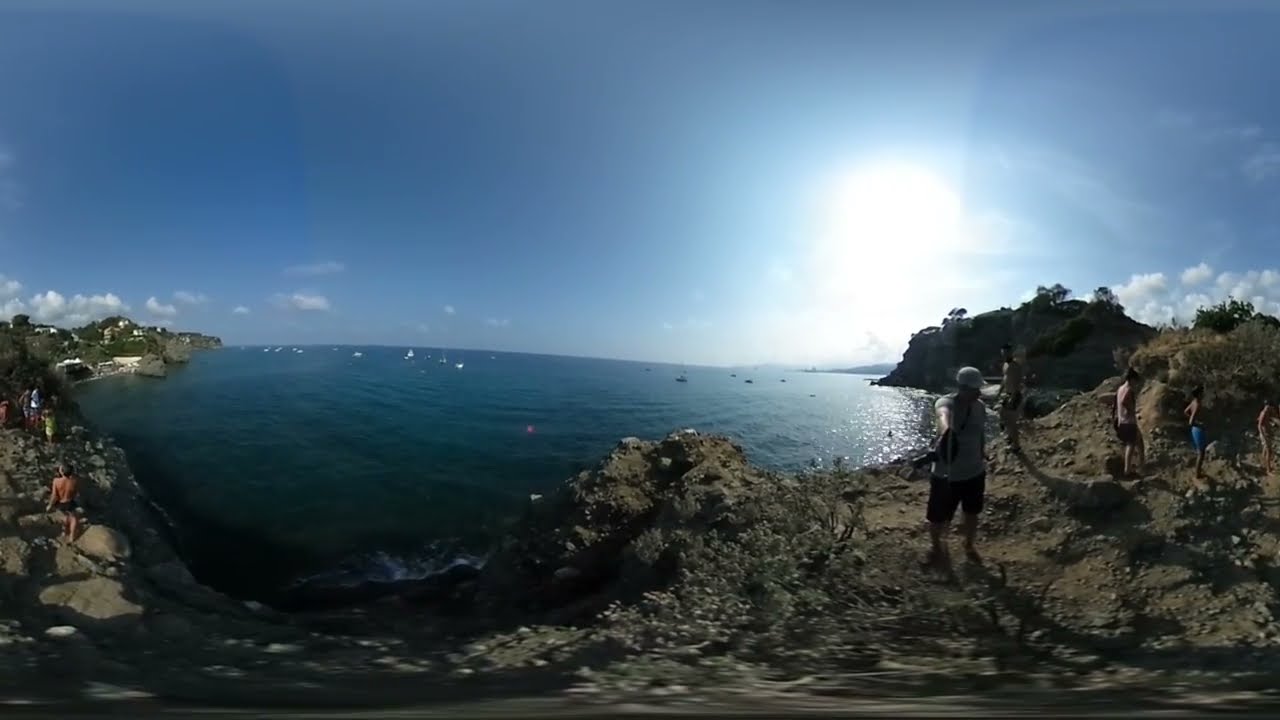The image captures a vibrant outdoor scene set along the shoreline of a vast, deep blue body of water, possibly an ocean, lake, or large river. The scenery is highlighted by a clear, bright blue sky scattered with a few puffy white clouds, bathed in the glowing light of the midday sun. The shore is a mix of tan-colored dirt and large, gray stone formations, creating a rugged, rocky landscape. 

On the right side of the image, several people are gathered, including a man wearing a white hat and black shorts, suggesting a relaxed day by the water. Among the group, some are shirtless, indicating casual, warm weather attire. Another individual, possibly holding a 360-degree camera, is present, indicated by the slightly distorted, panoramic view of the scene. 

In the background, high cliffs with green shrubbery descend dramatically to the water's edge on both the left and right sides. The horizon is dotted with several small sailboats and other watercraft leisurely moving across the water. Off in the distance, a quaint seaport town is visible, nestled among larger rock formations, adding a picturesque charm to the overall composition.